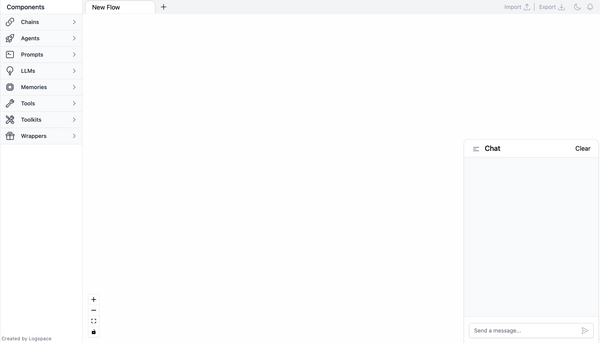The image is a screenshot of a web page or application interface with minimal information. The background is entirely white. In the bottom-right corner, there's a chat box interface. The chat box header is labeled "Chat," but the chat history is empty. Below the header, there's a text input field with the placeholder text "Send a message," indicating where users can type their messages. To the right of this field, there is a small arrow button used to send the message.

In the upper-left corner of the interface, there is a vertical menu labeled "Categories," featuring several expandable menu items. These categories include: Chains, Agents, Properties, LLMs, Memories, Tools, Toolbox, and Wrappers. Each category label has an arrow pointing to the right, suggesting that these are drop-down menus that expand to reveal more options when selected. For instance, selecting "Chains" would display all items nested under this category.